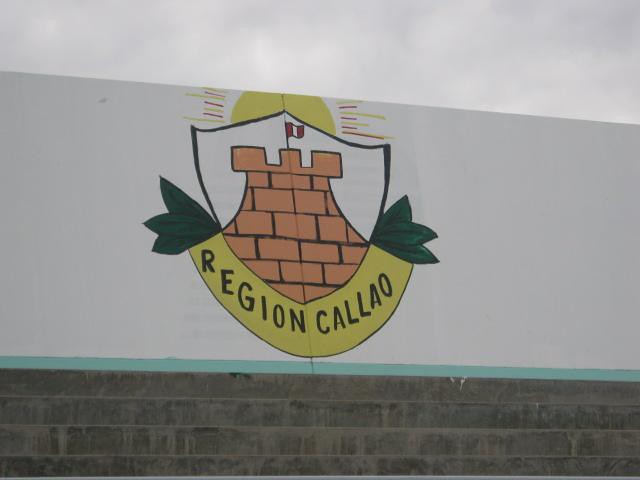The image captures an outdoor scene on a cloudy day, featuring a white wall with rows of gray bricks at the bottom. A mint green border separates the bricks from the central focus of the image—a distinctive sign. The sign prominently displays a crest outlined in black. This crest includes a depiction of a castle wall in the middle, topped with a red and white flag. Surrounding the crest are green leaves on both the left and right sides, while beneath it lies a yellow banner with the inscription "Region Kalau." In the background, a bright yellow sun is seen rising, adding a touch of vibrance to the composition.